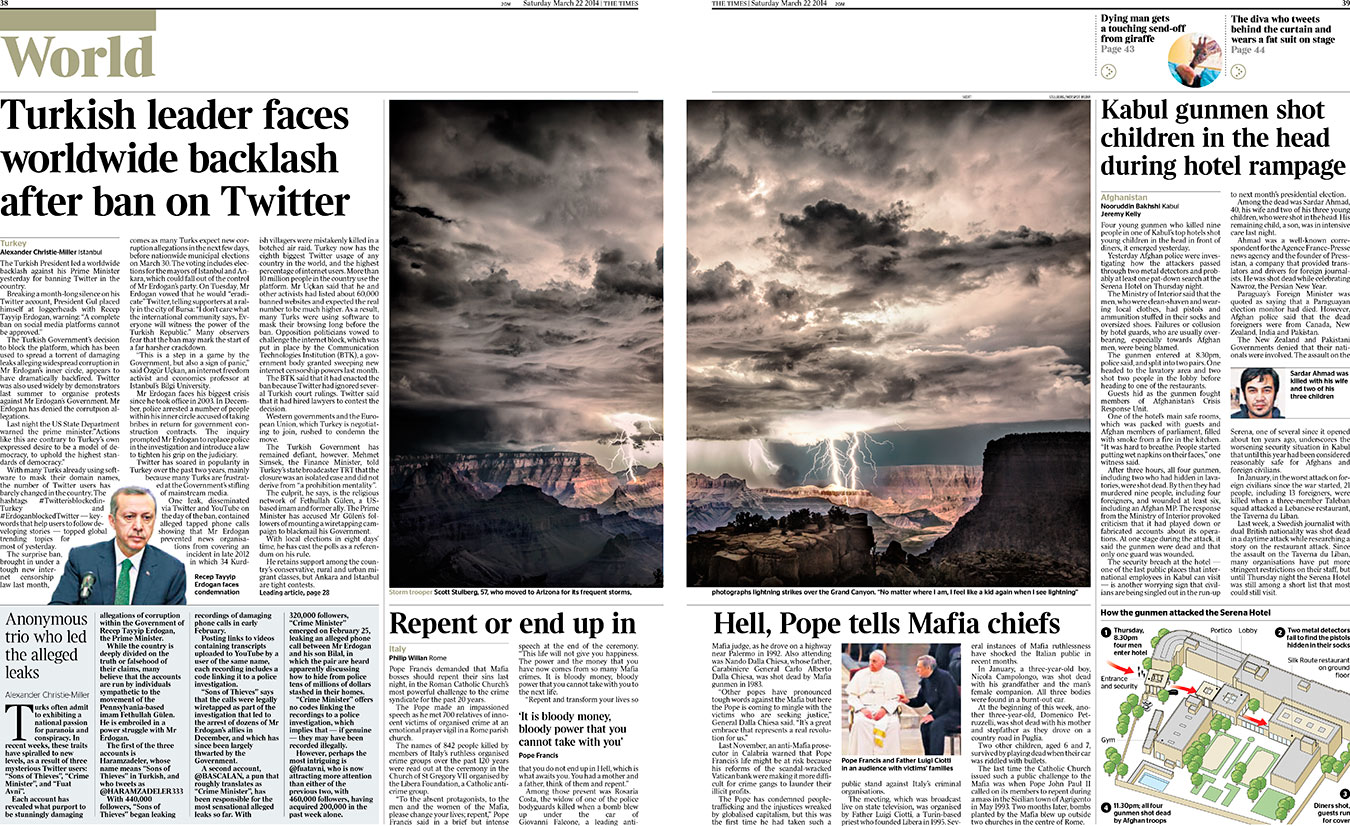The open magazine spread showcases two pages presented in a traditional newspaper format. The section title "World" is prominently displayed in the upper left corner, indicating coverage of global news.

Below the section title, a headline reads, "Turkish leader faces worldwide backlash after ban on Twitter." This article discusses the Turkish leader's controversial decision to ban Twitter in the country. An image positioned in the left middle of the page features a man in a dark blue suit and a green tie, potentially the Turkish leader, though his identity is not confirmed.

Dominating the center of both pages is a striking photograph reminiscent of the Grand Canyon. The image is dark and foreboding, with ominous clouds overhead and multiple lightning bolts striking the canyon floor, creating an intense visual impact.

To the right of this dramatic image, another headline captures attention: "Kabul gunmen shot children in the head during hotel rampage." This article describes a horrific incident of violence affecting young victims.

Further down on the left page, a partial headline reads, "Repent or end up in," but the remainder of the phrase is missing, leaving an ominous and open-ended message.

On the bottom center of the right page, a final headline declares, "Hell, Pope tells Mafia chiefs," indicating a stern ultimatum delivered by the Pope to Mafia leaders.